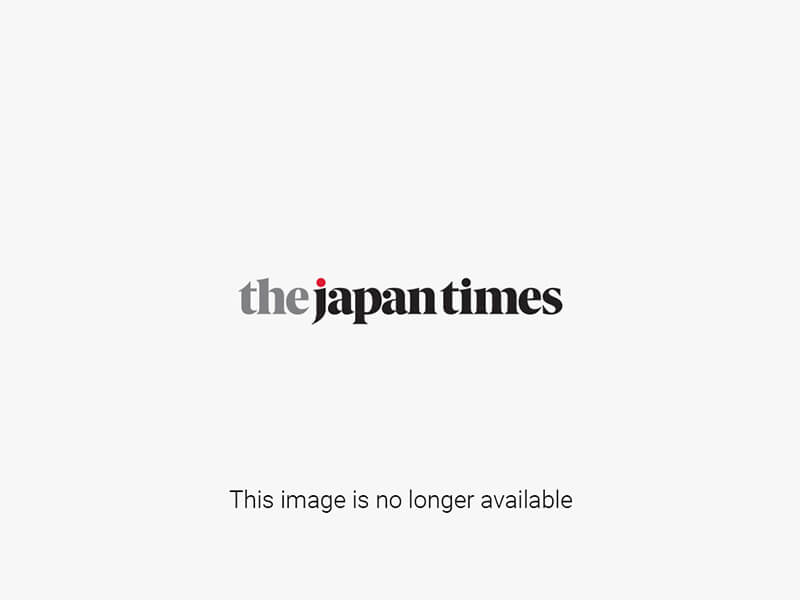This is an aerial view of a sprawling piece of farmland segmented into four sections, each with distinct characteristics. Encircled by a country road that curves around it, the landscape features a variety of agricultural states: the top left section displays lush crops, adjacent to a brown strip of mowed land with dried grass. Moving clockwise, the next section is a densely packed verdant rectangular field of thriving crops. To its right, the upper segment shows freshly tilled dark soil. Running through all four sections, an irrigation culvert facilitates water distribution across the farm.

Surrounding the segmented fields are patches of vegetation, including tall cedar trees and unkept grass. In the left corner of the image, on the opposite side of the road, there is a noticeable farmhouse with an attached barn. This barn has a distinctive façade, half painted white and the other half aged to an ash-gray hue. Next to this main structure is a smaller white building, possibly another barn or shed, contributing to the rustic charm of this country scene. Above, telephone lines stretch across the landscape, adding to the rural ambiance. The overall image captures a sunny day, highlighting the vibrant and varied textures of the farmland.